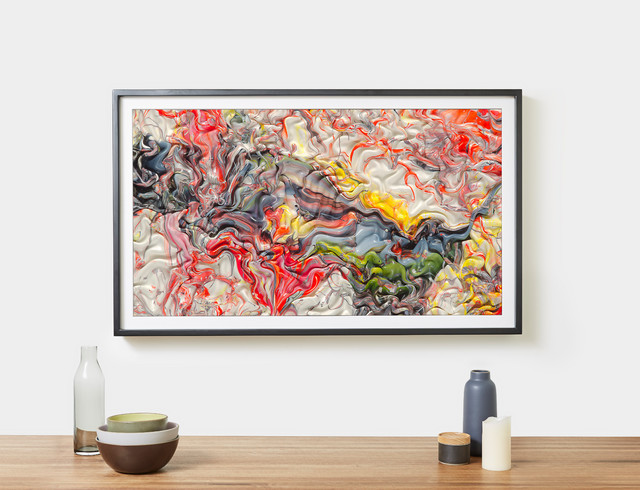The image features a painting hanging on a stark white wall. The painting is framed in a black frame with a white matting that borders the rectangular artwork. The dynamic painting is a chaotic blend of squiggly and smooth flowing lines, giving it a textured and layered appearance, with thick applications of paint. Predominantly, the composition includes white lines reminiscent of intestines intersected with drips of blue paint. The center bursts with a mixture of yellow, black, and red lines, while the upper left corner darkens with deeper black shades. Contrastingly, the right side features yellow streaks and the bottom corners of the painting amalgamate all the colors, with the upper right corner displaying mostly red hues.

Beneath the painting, there is a brown wooden table. On the left side of the table, there's a clear plastic bottle and in front of it, three bowls are stacked: a brown one on the bottom, a gray one in the middle, and a light green one on top. To the right of this arrangement, there is a gray water bottle. In front of it, there is a small black container with a brown cap and next to it, a white candle. The overall scene is a blend of abstract artistic expression and everyday objects, providing a striking contrast between the vibrant, chaotic painting and the sober, utilitarian items on the table.